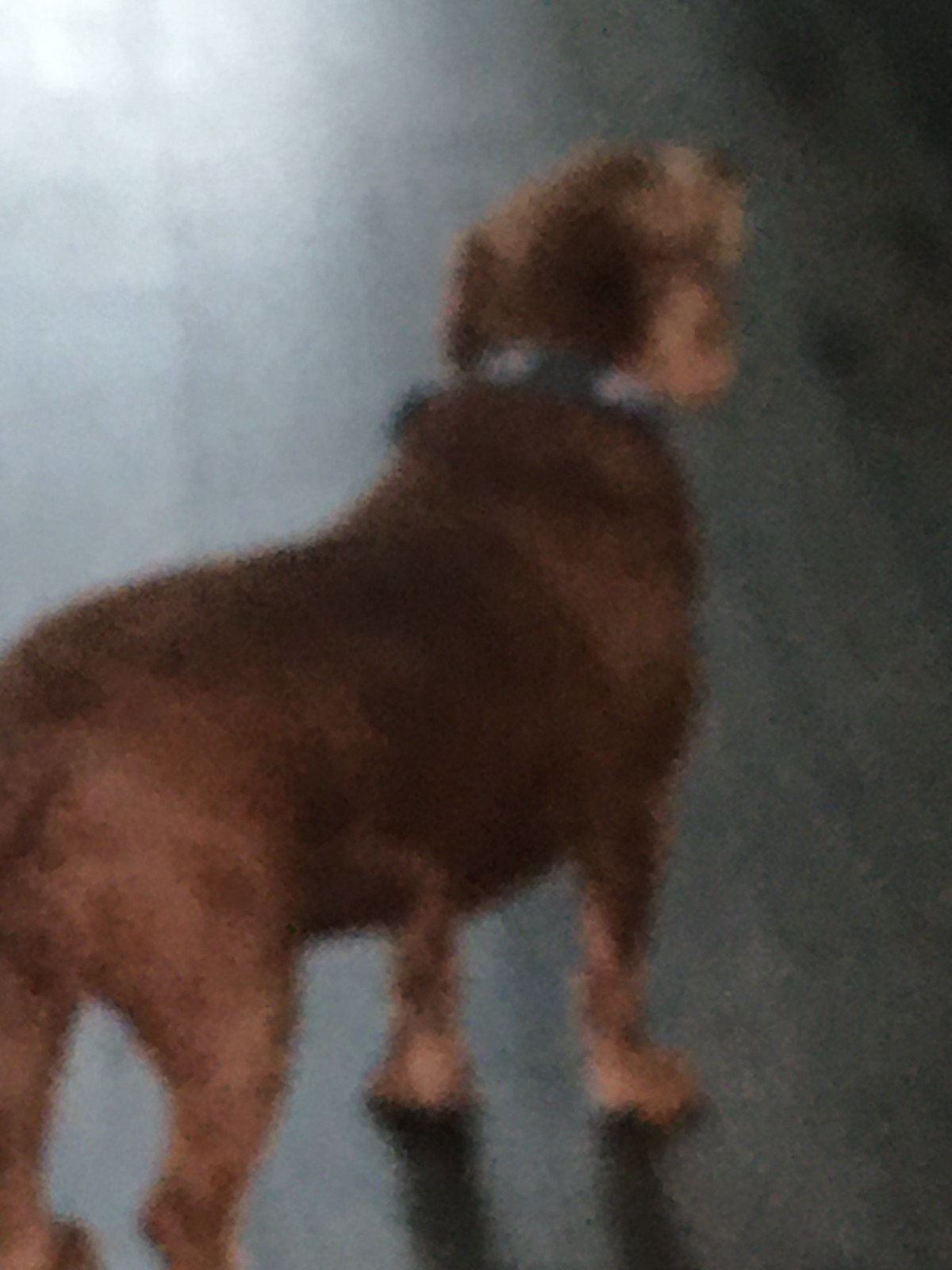A blurry image depicts a short brown dog standing indoors, seemingly in the middle of a house. The dog, facing the right side with its backside prominently visible, has a blue collar with white writing. The dog’s coloring transitions from a predominantly dark brown body to lighter brown hues on its front face, ears, and underside of its front paws which also feature some white markings. Light enters from the top left corner, illuminating the gray floor and creating a contrast with the dark area in the top right corner. The setting feels cozy and indoors, accentuated by the light variation and the visible details of the dog's coloring and collar.